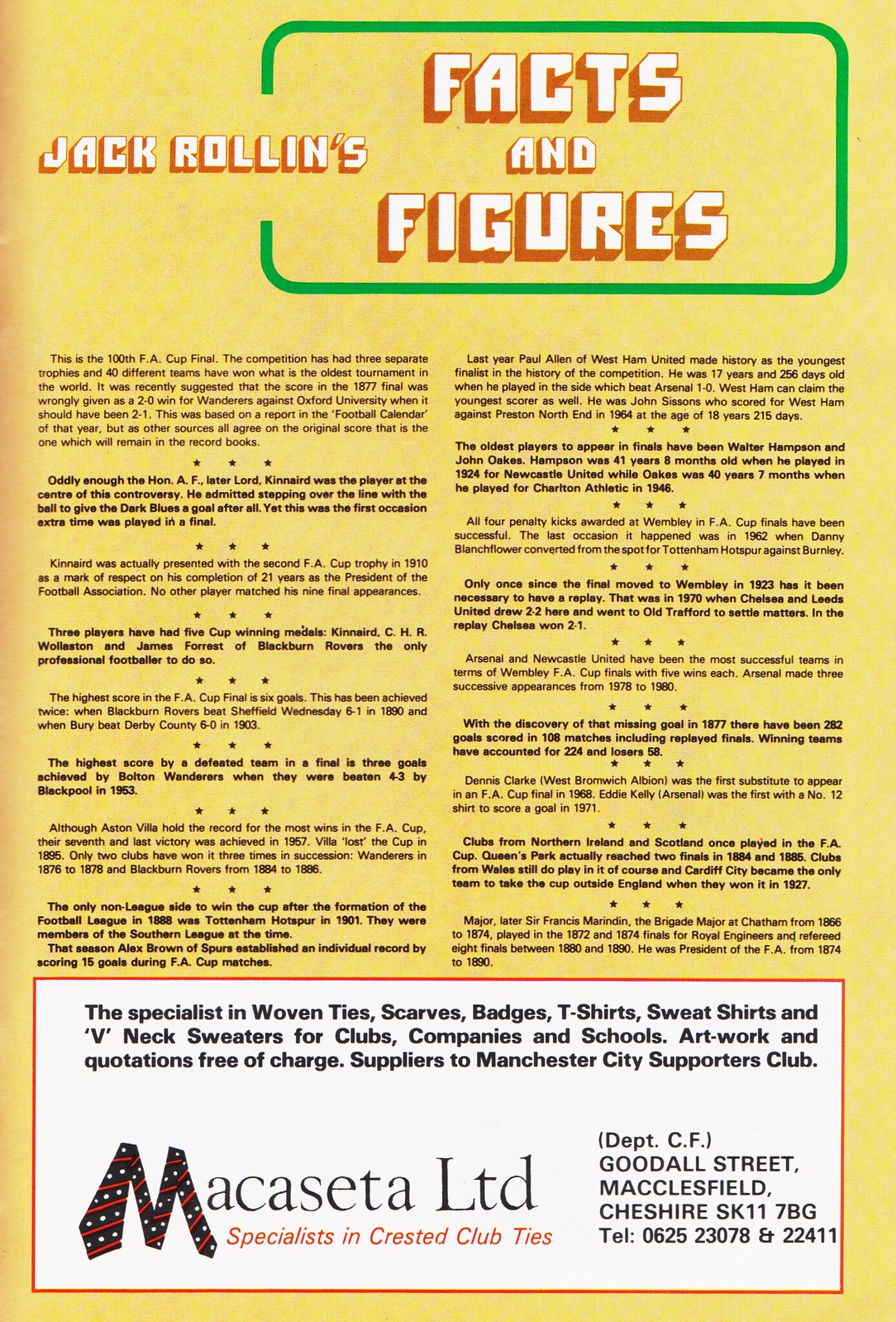The image features a predominantly yellow background titled "Jack Rowlands' Facts and Figures," with the title set in large white letters highlighted in orange and encircled by a green rectangular outline. This title takes up about one-fourth of the top portion of the view. The main content comprises roughly eighteen small black paragraphs, divided by three little dots, spanning the center of the image. These text passages, rich with historical anecdotes and trivia, detail various facts such as the 100th FA Cup Final, the controversy around the 1877 final score, and the role of Lord Kinnaird in early football history. Below these paragraphs lies a white rectangle outlined in red, which contains an advertisement. This ad is for "Makasseta Ltd.," specialists in woven ties, scarves, badges, T-shirts, sweatshirts, and V-neck sweaters for clubs, companies, and schools. It includes a tagline offering artwork and quotations free of charge, and cites their association with Manchester City Supporters Club. Additionally, it features larger text promoting their crested club ties, along with the address, phone number, and a distinctive logo where the 'M' is designed to resemble a tie.